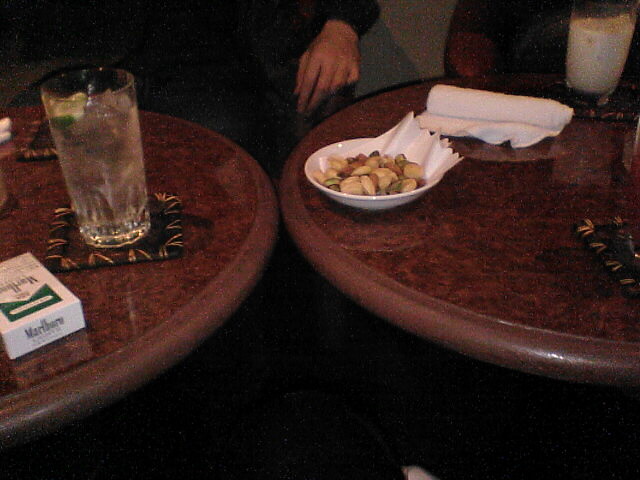This color photograph, taken in a landscape orientation, captures a detailed view of two identical, circular wooden tables with a glossy walnut finish, placed side-by-side in what appears to be an indoor pub or restaurant setting. The table on the left features several items: in the bottom left corner, there's a box of Marlboro cigarettes, distinguishable by its white color and forest green strip with the brand name in black serif font. To its right, a clear glass filled almost to the rim with clear liquid, ice cubes, and a lime wedge rests on a black square coaster. Behind these items is a person's hand, partially visible at the top center of the image. On the table to the right, there's a white ceramic bowl filled with beige and green items that look like mixed nuts or dried fruits, along with a rolled-up white napkin. Another clear glass, this one filled with a cream-colored liquid, is situated at the top right corner of the table. This meticulously detailed scene gives a convincing impression of a casual dining setting.